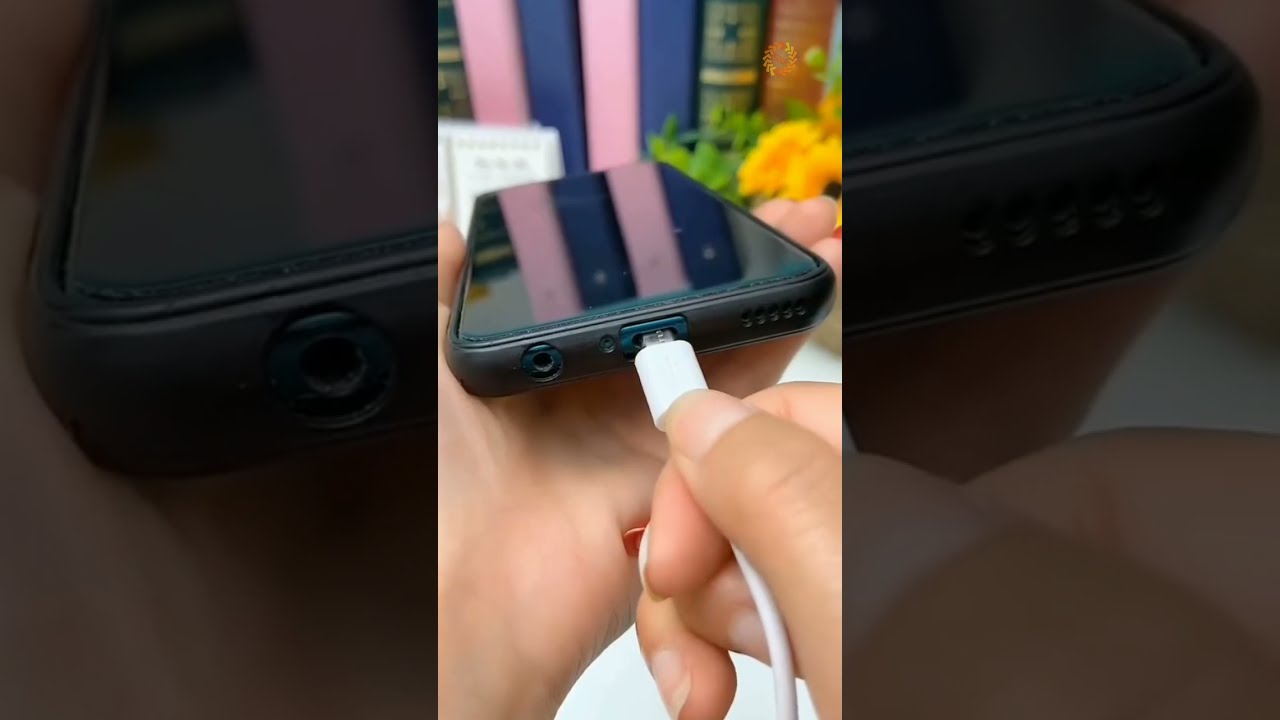This image is a horizontally arranged composition featuring a central close-up of a black cell phone being held by a person with brown skin. The person is inserting a white charging cable into the phone's port using their right hand, while their left hand supports the phone. The backdrop is somewhat blurred but reveals an indoor setting, likely a bookshelf, with an array of books in various colors, including pink, blue, green, and orange. Flanking the central image are darker, blurrier close-up views of the left and right sides of the phone, with the right side also showing part of the fingers holding the device.